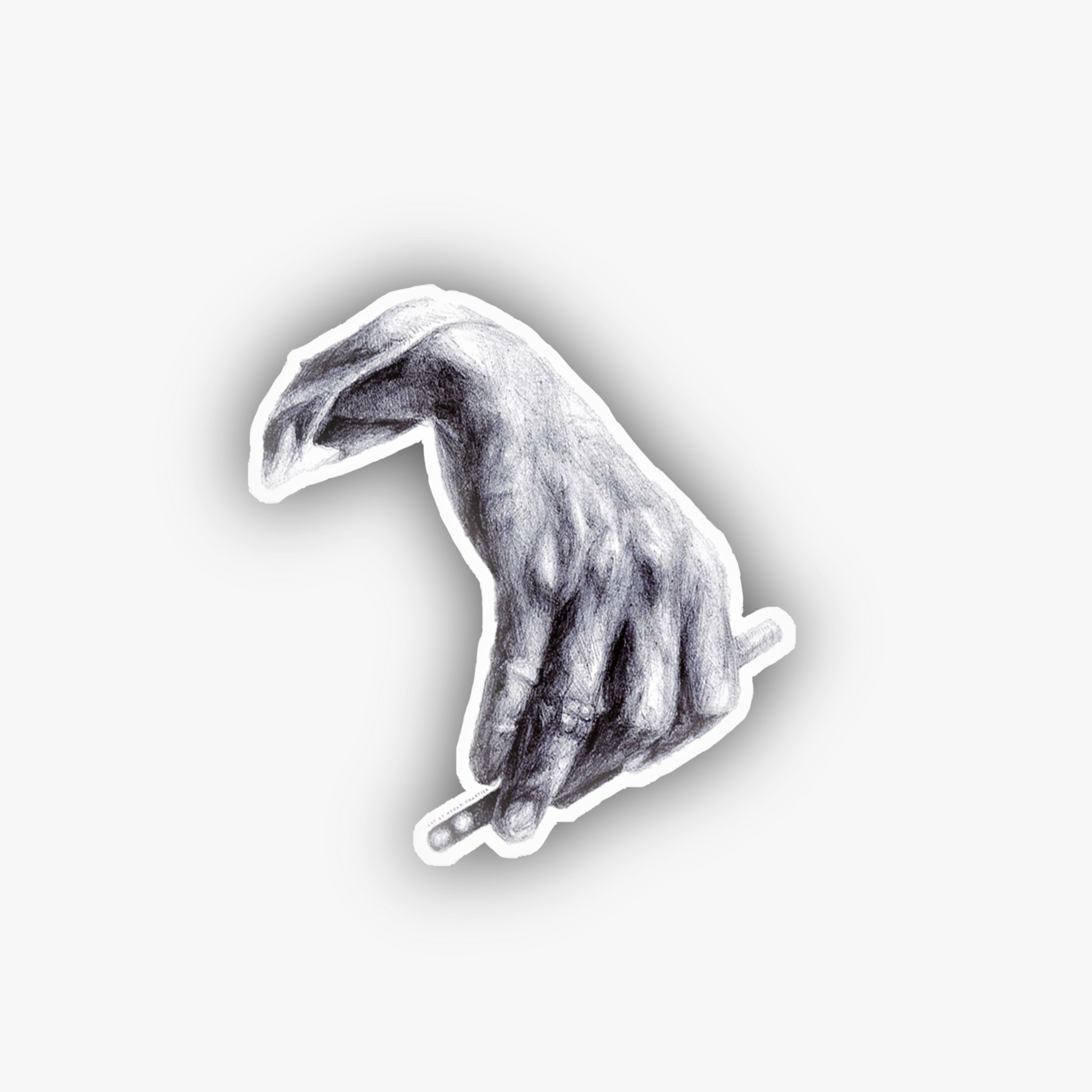This is a detailed black and white pencil drawing of a limp-wristed hand delicately holding a pencil. The highly detailed hand, emerging diagonally from the top left to the bottom right, features visible knuckles, veins, and wrist bone, adding a realistic touch to the image. The presence of a ring on the third finger and the subtle sleeve of what appears to be a robe around the wrist enhance the hand's delicate and precise appearance. The image is set against a grey background, outlined in white with a shadow effect around the entire drawing, creating a three-dimensional look. The meticulous shading on the fingers, fingernails, and entire hand highlights the shadows and dimensions, making the drawing appear almost lifelike.